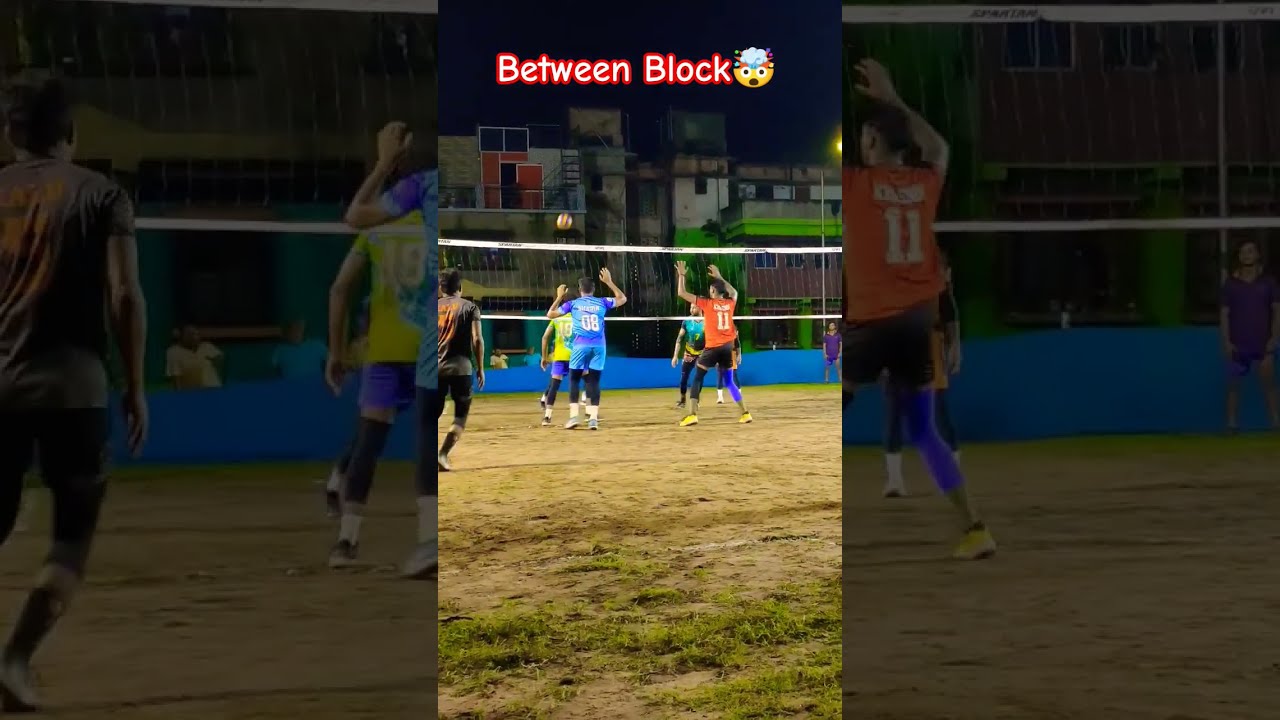This horizontal rectangular image captures a group of young men intensely engaged in a game of volleyball in an urban setting. The focal point is a vertical rectangle in the center featuring the text "BETWEEN BLOCK" in white letters outlined in red, accompanied by an exploding head emoji. The scene is set against a backdrop of rundown, multi-colored buildings, some with neon green and orange paint, while others remain bare concrete. A blue fence runs along the base of these buildings. 

In the mid-ground, a white volleyball net with black webbing stretches horizontally from left to right, delineating the playing area. The players, clad in vibrant athletic gear reminiscent of soccer attire, include a man in an orange jersey with the number 11, another in a blue jersey with the number 08, and a third in a yellow jersey numbered 19. The remaining players, whose numbers are not visible, also sport various colored kits, including blue and black shorts.

The ground beneath them is a mix of dirt and sporadic patches of green grass and weeds, indicating a poorly maintained field. Adding depth to the image, the left and right sides feature faded close-up shots of the players positioned on their respective sides of the central picture, creating a dynamic and layered visual effect.